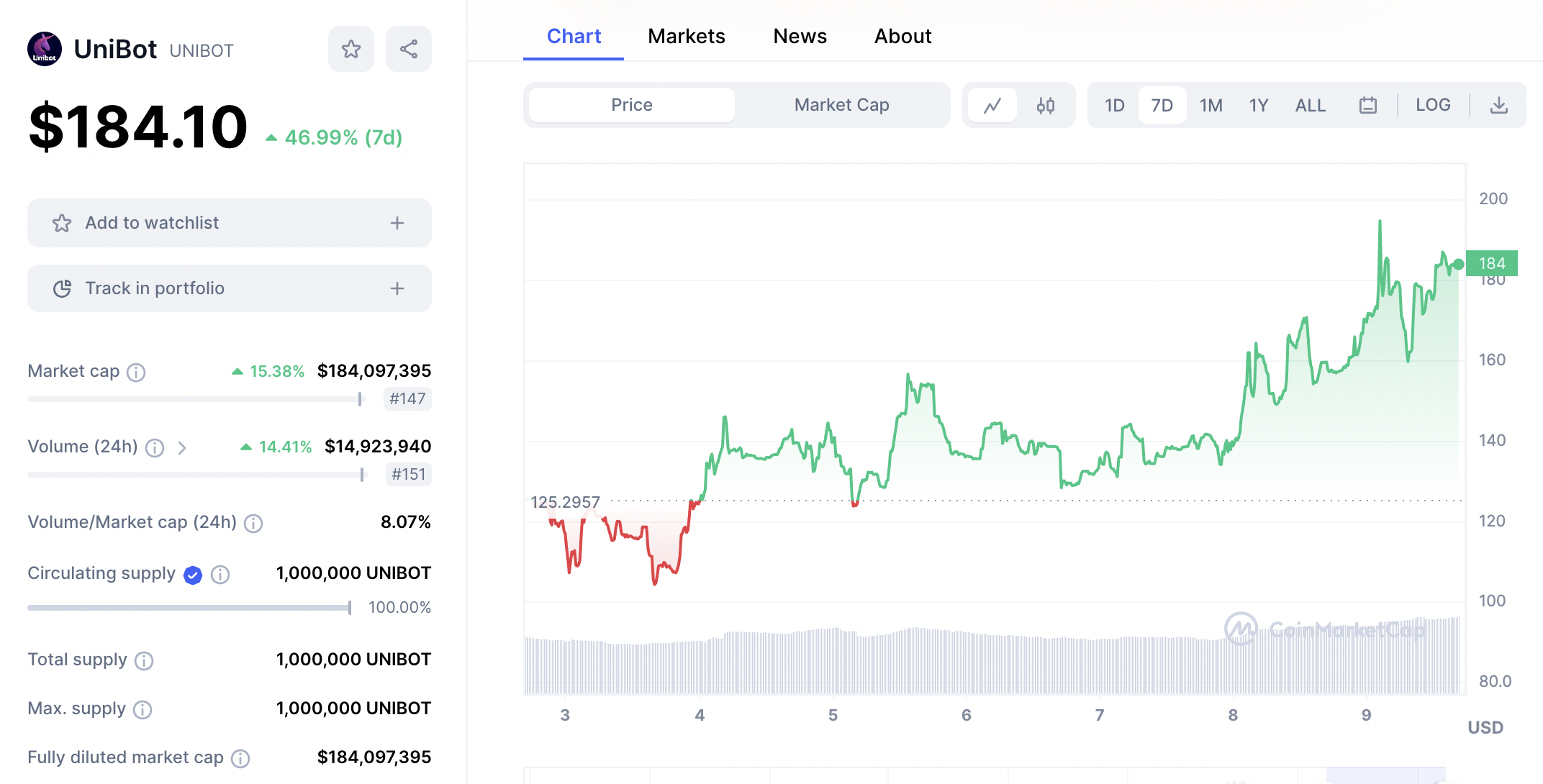### Detailed Description Caption: 

The screenshot depicts a dynamic and information-rich webpage dedicated to stock market analysis. The layout is predominantly split into two main sections.

**Left Section:**
- **Title and Controls:** The top-left corner showcases the name "Unibot" twice; first in black bold letters accompanied by an avatar on the left, and then in non-bold all capital letters on the right. 
- **Interactive Buttons:** Adjacent to the title are two square buttons with rounded corners—one featuring a star icon and the other a share icon.
- **Stock Price:** Below these buttons, the stock price is prominently displayed in large black bold numerals reading "$184.10."
- **Price Change:** Underneath the price, small green text with an upward arrow indicates a recent change: "$46.99 7D."
- **Action Buttons:** Two options are available for user interaction: "Add to Watch List" and "Track Portfolio," each illustrated with relevant icons and housed within a gray rectangular area with rounded corners and a plus sign on the right.
- **Additional Info:** Further down are multiple rows of detailed financial metrics:
  - **Market Cap:** Listed with an information icon, showing "15.38%" and "$184,097,395."
  - **Volume (24 Hours):** Presented with an info icon and a greater-than symbol, featuring "14.41%" in green text alongside "$14,923,940."
  - Further rows contain similar detailed metrics, separated by thin gray lines for clarity.

**Right Section:**
- **Graphical Representation:** Dominating the right side is a comprehensive graph:
  - **Color-Coded Data Line:** The graph initiates in red below the 120 line, transitions to green as it surpasses this threshold, briefly dips back into red, and concludes in green near the 184 mark.
  - **Y-Axis Labels:** Numerical labels are on the right, from top to bottom, in ascending increments of 20: "200, 180, 160, 140, 120, 100."
  - **X-Axis Labels:** Range from "3" to "9," indicating data over a span of time.
  - **USD Label:** Located at the bottom right corner signifying the currency.
 
At the top of this section, four navigational tabs are visible:
- **Tabs:** "Chart" is selected, highlighted in blue with an underline, while the other tabs include "Market," "News," and "About."
- **Filters and Buttons:** Two filters— for price or market cap—and additional buttons are situated to the far right.

This well-structured and visually engaging layout succinctly conveys crucial stock-related information alongside interactive elements for user engagement and further exploration.